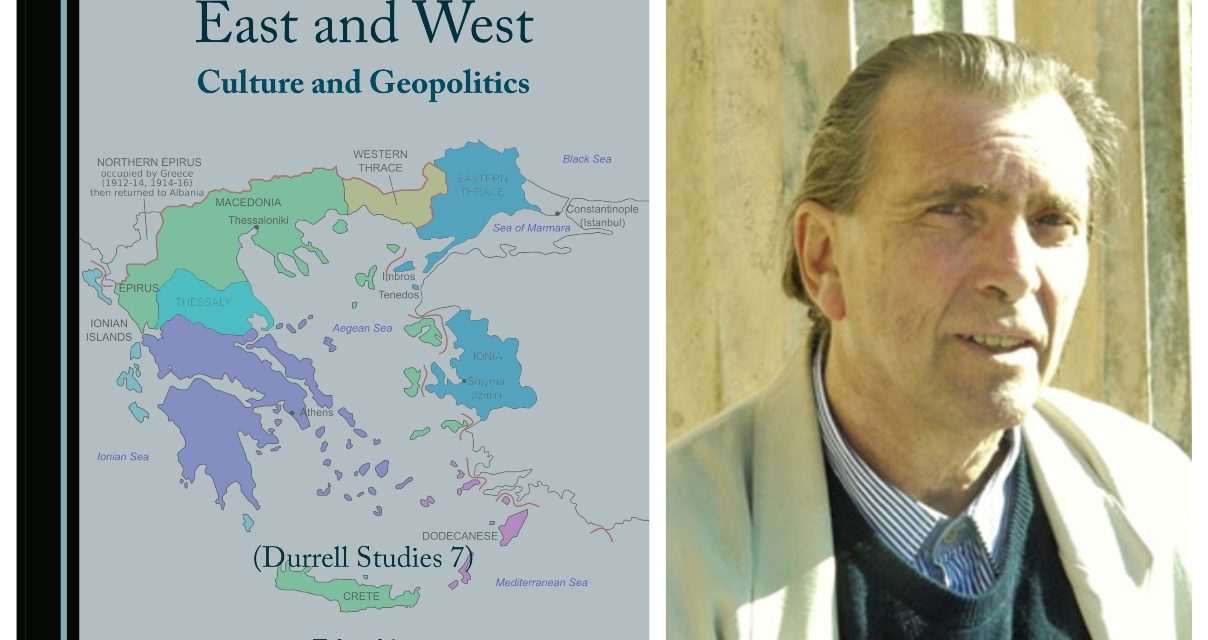The image is split into two sections. On the left is a map titled "East and West: Culture and Geopolitics," highlighting various regions including Northern Epirus, Western Thrace, Black Sea, Sea of Marmara, Aegean Sea, and Mediterranean Sea. The map features areas colored in blue, purple, green, and yellow, and includes the text "Durrell Studies" and the number 7. On the right side stands a man with brown hair slicked back, giving a slight smile while squinting in the bright sunlight. He is dressed in a light tan vest over a blue and white collared shirt, complemented by a grey sweater. The background appears to be an outdoor setting with a wood fence and some green and tan elements. Shadows cast across his jacket further emphasize the sunny day.